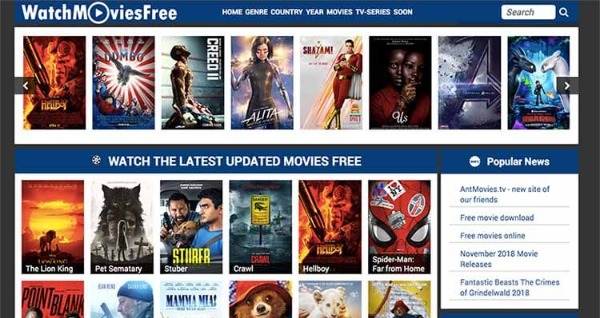This detailed caption describes a website interface for streaming movies:

---

This is a screenshot from a movie streaming website featuring a sleek gradient background transitioning from blue to black. Positioned in the upper left corner, "Watch Movies Free" is displayed prominently in white font, with the 'O' in "Movies" cleverly designed as a play button. Directly below this text lies a row of movie thumbnails available for free viewing. The list begins with "Hellboy," followed by "Dumbo," "Creed 2," "Shazam," "Us," an icon with the letter 'A' which likely represents "Avengers," and "How to Train Your Dragon."

Above the row of films is a navigation bar with the following options: "Home," "Genre," "Country," "Year," "Movies," "TV Series," "Soon," and a search feature. The search bar comprises a white rectangular field with the word "Search" in black font, accompanied by a white magnifying glass icon to its right.

Below the row of available movies, a blue rectangle holds the text "Watch the Latest Updated Movies Free" in white font. Further down, the section is labeled "Popular News," followed by another listing of films including "The Lion King," "Pet Sematary," and "Stirrer."

---